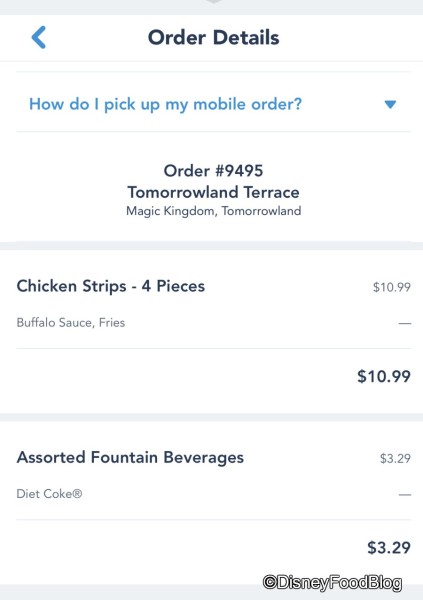This is a detailed smartphone screenshot from the website Disney Food Blog. At the top of the screen, there's a section titled "Order Details" with a left-facing arrow on the left side. Directly below, there's a question, "How do I pick up my mobile order?" accompanied by a drop-down arrow on the right.

The order number 9495 is listed next, followed by the location specifics: Tomorrowland Terrace in Magic Kingdom's Tomorrowland. The order consists of the following items: chicken strips (four pieces) priced at $10.99, buffalo sauce fries also priced at $10.99, and assorted fountain beverages at $3.29. Below the assorted beverages, Diet Coke is listed with its registered trademark icon and logo, and next to it, a line without a price.

The subtotal for the assorted fountain beverages is $3.29. At the bottom of the screenshot, the caption reads 'Disney Food Blog' as a single word followed by the copyright symbol. This screenshot clearly summarizes the order details and includes a prompt for picking up the mobile order along with the order number.